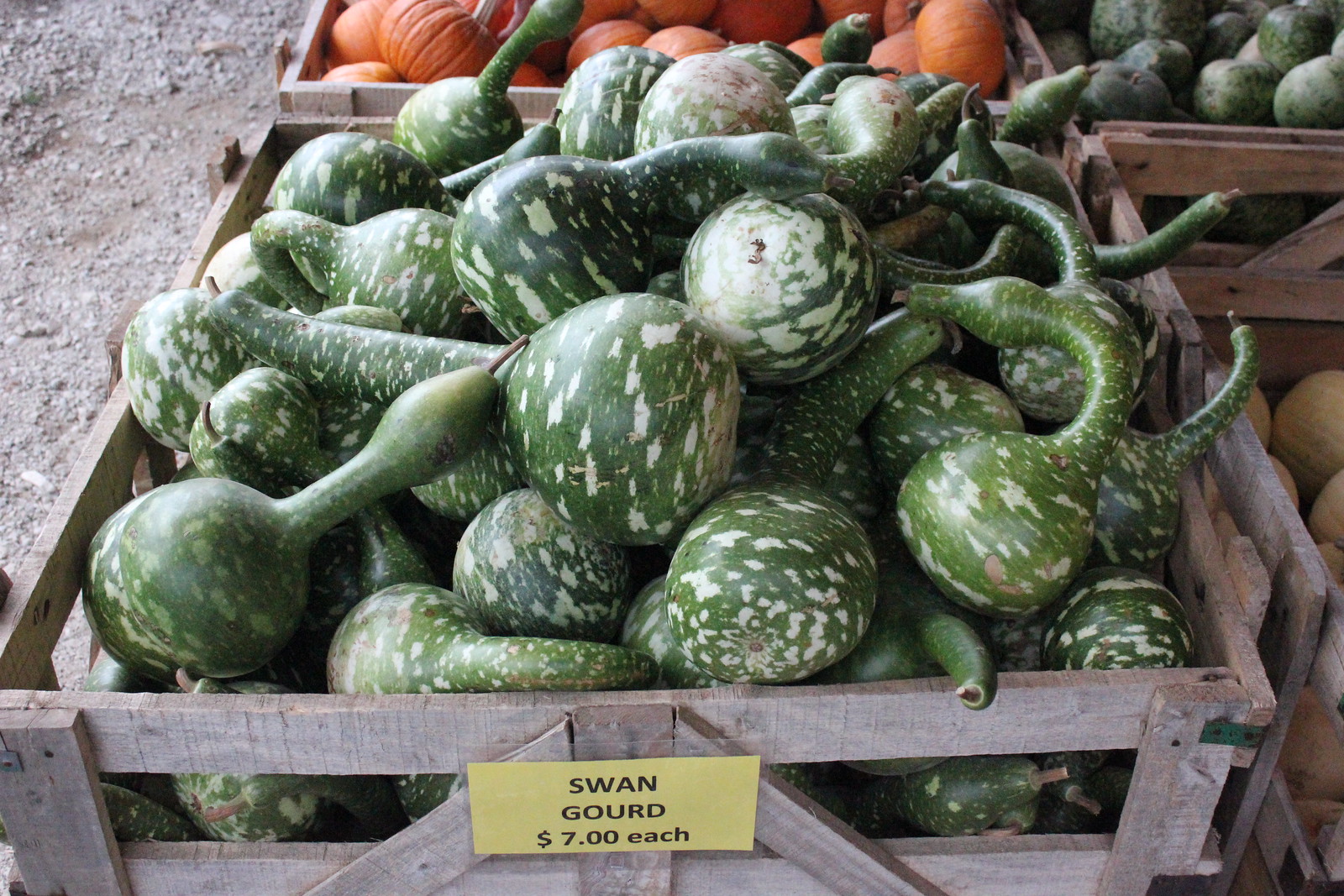The image depicts an outdoor scene, reminiscent of a lively farmer's market, with three weathered wooden crates arranged on a dirt and gravel ground. The most prominent crate, positioned at the bottom center and filling the frame, is brimming with at least 50 green swan gourds, each adorned with distinct white spots. These gourds have curved and straight stems, lending them their namesake with a bulbous end and a slender arched neck. Attached to this crate is a yellow rectangular sign in black ink that reads "swan gourd, $7 each." Adjacent to this crate, partially visible and slightly cut off, is another wooden crate filled with small, circular orange pumpkins, identifiable by their prominent stems. The background reveals an additional crate, though its contents are not clearly discernible due to it being mostly out of frame. To the left, the ground is visible, strewn with dirt and small pebbles, adding to the rustic and earthy ambiance of the market setting.